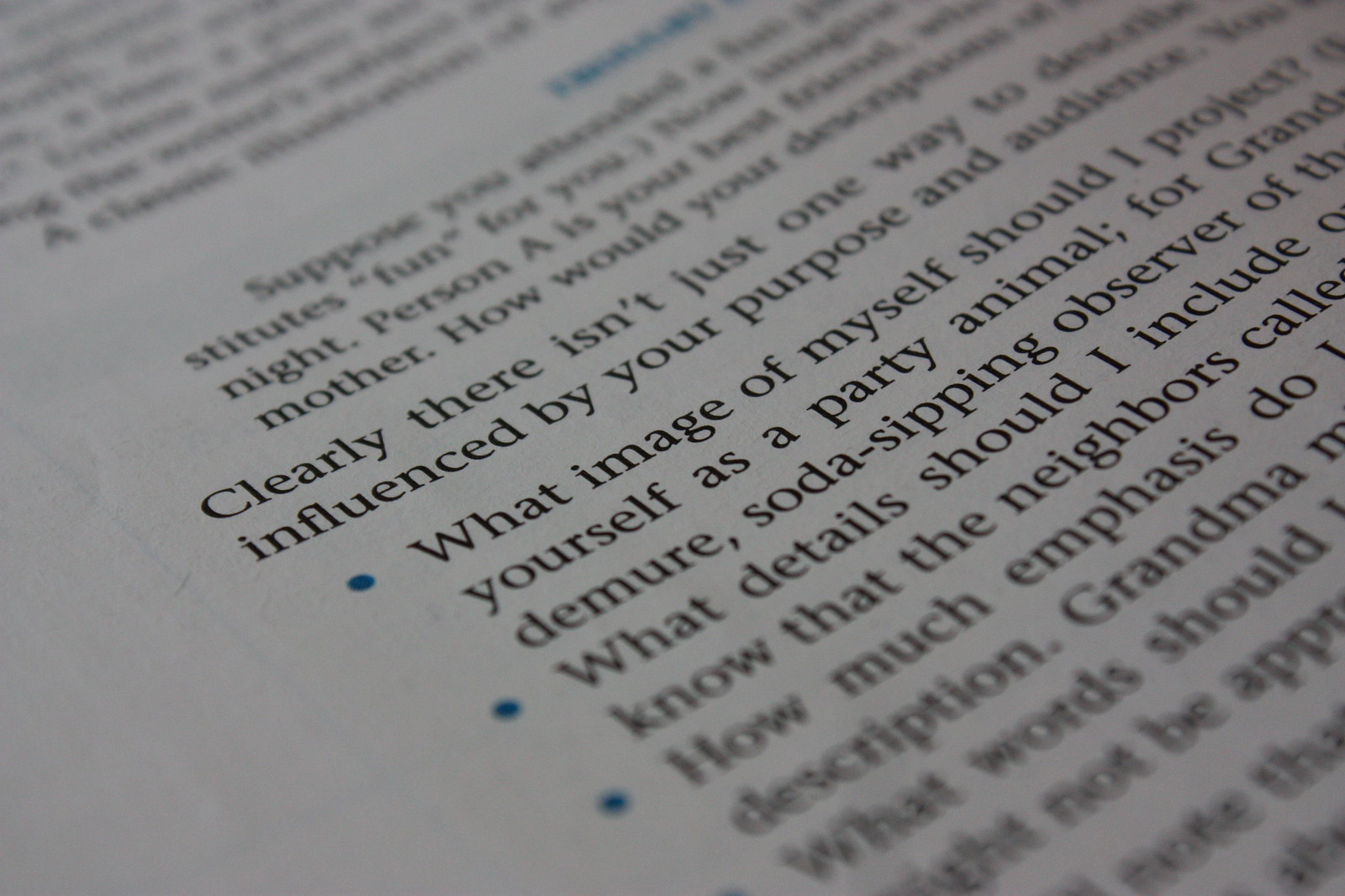The image is a close-up photograph of a white page filled with black text, appearing to be a piece of paper or a book page. The photograph is taken with a strong depth of field, causing the text to become progressively blurrier outside of a central horizontal band. The page is displayed diagonally from left to right. The visible, readable text includes phrases such as "Clearly there isn't just one way to… influenced by your purpose and audience… what image of myself should I project… yourself as a party animal for grand demure soda sipping observer… what details shall I include… know that the neighbors called how much emphasis…". There are a few bullet points under the readable text. The overall color scheme of the image includes black, white, and some hints of blue.